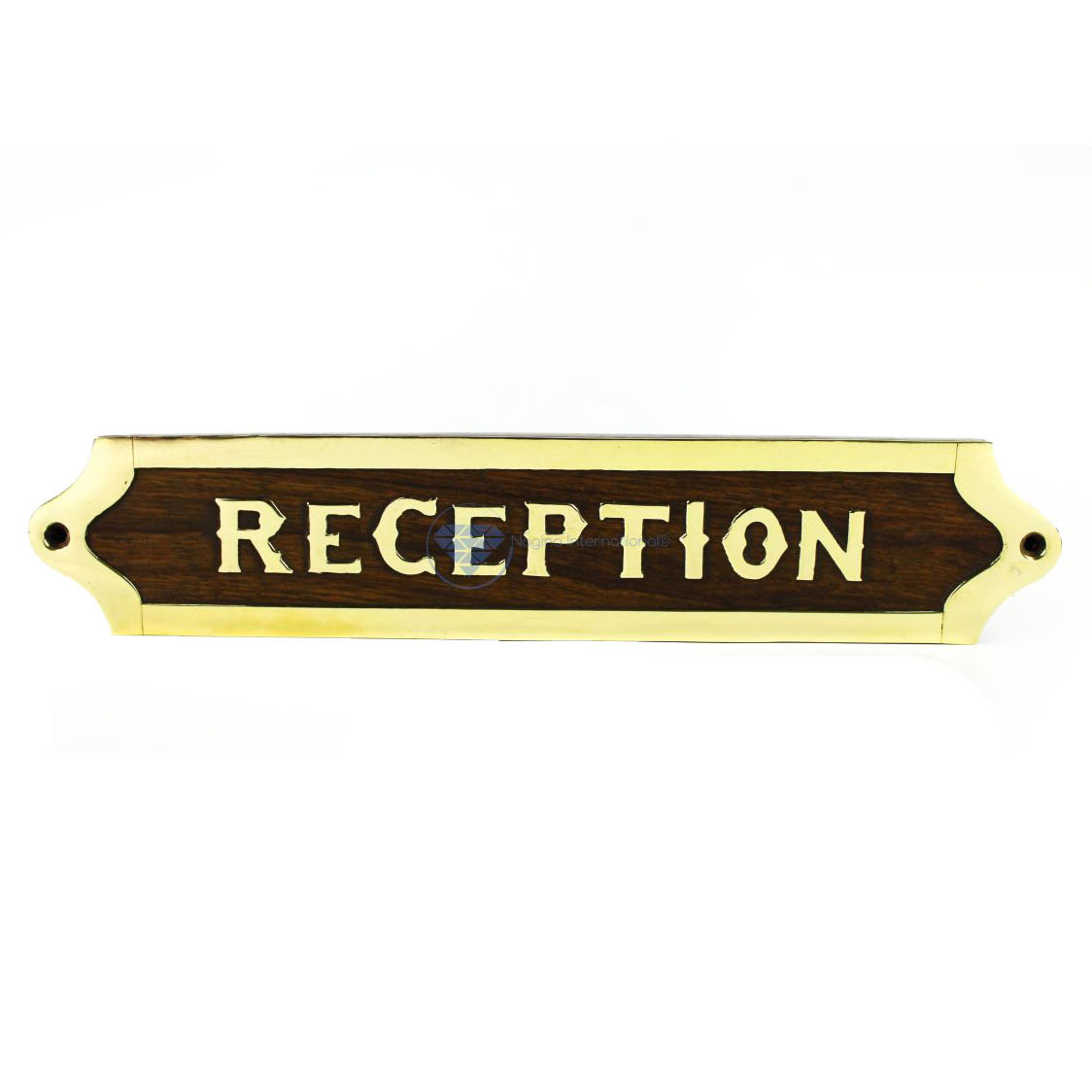This is an image of a rectangular sign, likely a plaque on a wall, indicating the reception area of a hotel, lodge, or bed and breakfast. The sign is made of brown wood with a brass border featuring slight curves at the top edges and straight lines at the bottom. There are two holes on either side of the sign for attaching it securely to the wall with screws or nails. The word "RECEPTION" is written in large, all-capital brass letters centrally positioned on the plaque. The font style is somewhat old-fashioned, adding a quaint charm to the sign. Notably, above the second "E" in "RECEPTION," there appears to be a diamond-shaped watermark or copyright symbol in light blue, composed of small triangles and encircled. The brass border has aged, giving parts of it a slightly yellowish hue, suggesting that it has been in place for quite some time.